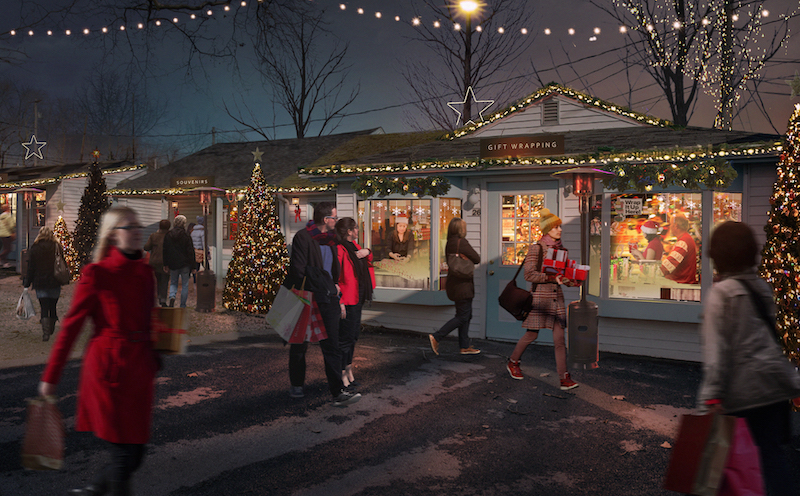This nighttime outdoor photo, likely taken during Christmastime, captures a lively small-town holiday scene. The foreground features a well-lit wooden chalet store with the sign "Gift Wrapping" on its roof, indicating a festive atmosphere inside where people don Santa hats. Shoppers, predominantly around the age of 30, fill the streets, warmly dressed in coats, scarves, and hats, carrying bags which suggest they've been shopping. The quaint town's numerous standalone shops are adorned with strings of colorful lights outlining their roofs, enhancing the festive ambiance. Decorated Christmas trees, some topped with stars, and illuminated bare winter trees further add to the holiday spirit. In the background, a visible tree line with no leaves adds to the wintry feel, while the moon shines down, providing a serene backdrop. The cheerful shoppers and illuminated decorations together evoke the joyous essence of Christmastime.